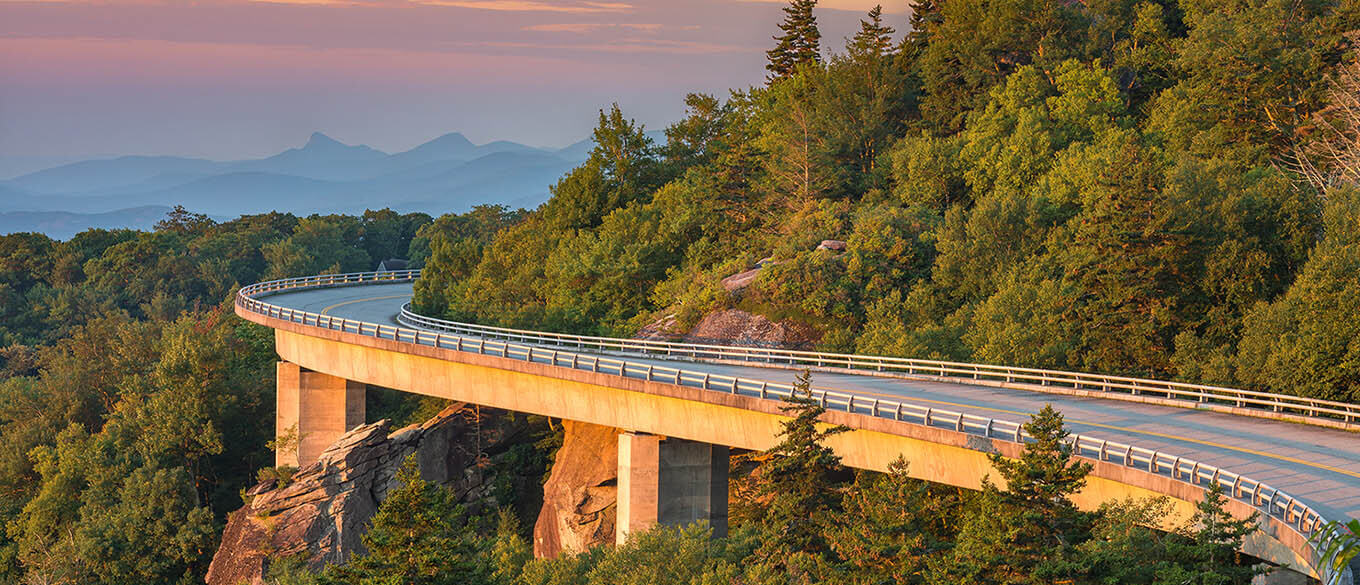The photo captures a stunning outdoor scene during what appears to be either early morning or dusk, featuring a winding highway that curves along the side of a mountainous terrain. The highway, an elevated bridge held up by large concrete pillars, starts at the bottom right corner of the image, crosses to the middle, and then curves back to the right, gradually disappearing behind the lush, tree-covered mountain. The rocky mountainside beneath the bridge contrasts with the dense greenery, adding texture to the landscape. In the far distance, a majestic mountain range looms, painted in hues of dark blue. The sky above is hazy and softly illuminated in a palette of light blue, pink, and purple, suggestive of the sun either rising or setting. The bridge itself is gray with both a thin yellow line and a white center divider running down its middle, and it is gently lit by the ambient light of the serene sky.